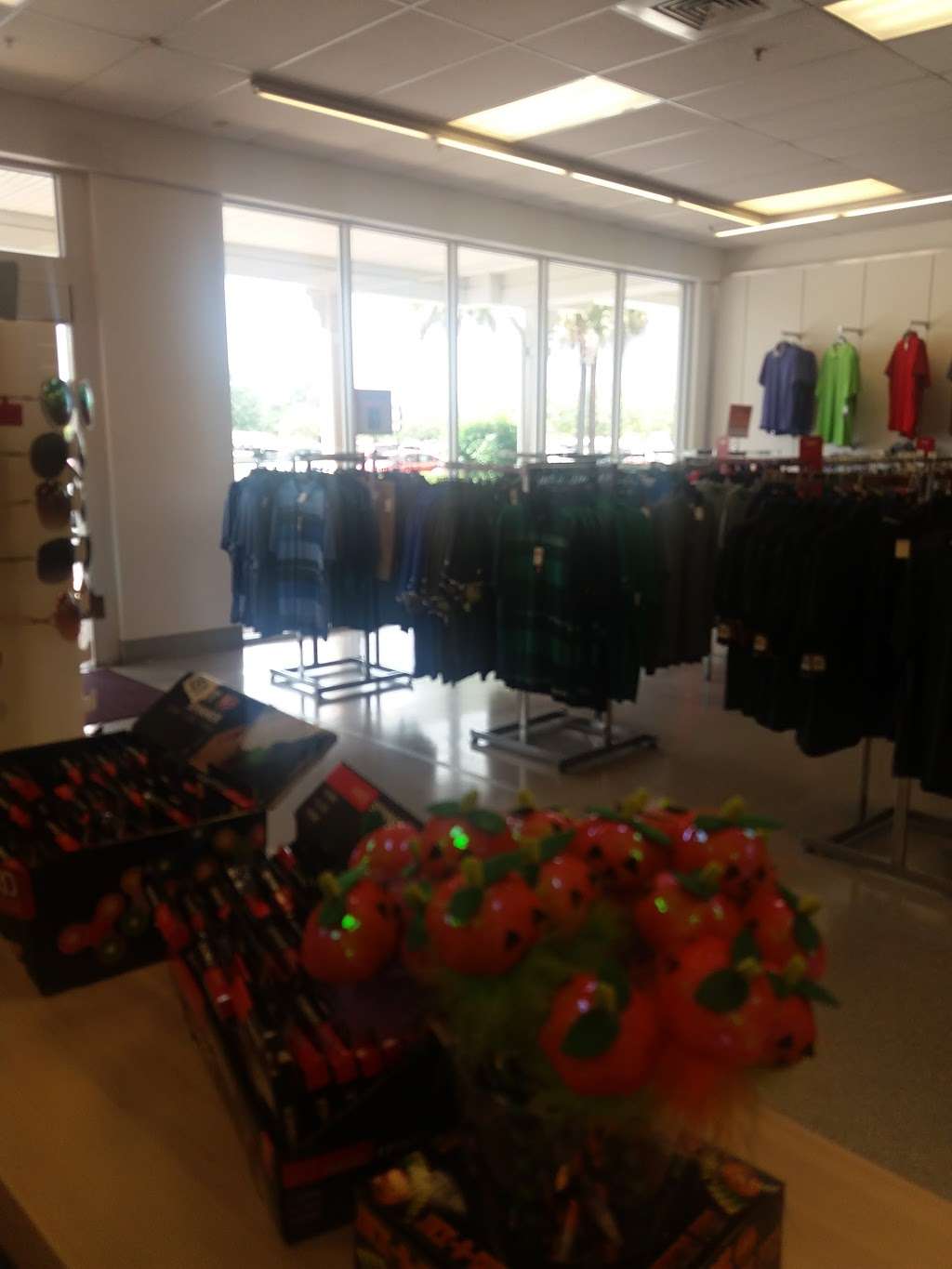The image depicts a clothing store interior featuring several aisles of metal clothes racks filled with various garments. At the back, there is a five-pane window framed by an off-white wall, from which hang shirts in shades of blue, green, and red. In the foreground, on a brown countertop, sit what appear to be red items in boxes alongside another box that is black and red in color. The ceiling consists of white square foam panels with fluorescent lights that illuminate the space. The floor appears to be made of marble. To the right of the five-pane window is a white partition, with hats possibly hanging from it. Additionally, there is a small window situated at the top left side of the store, augmenting the natural light in the room.